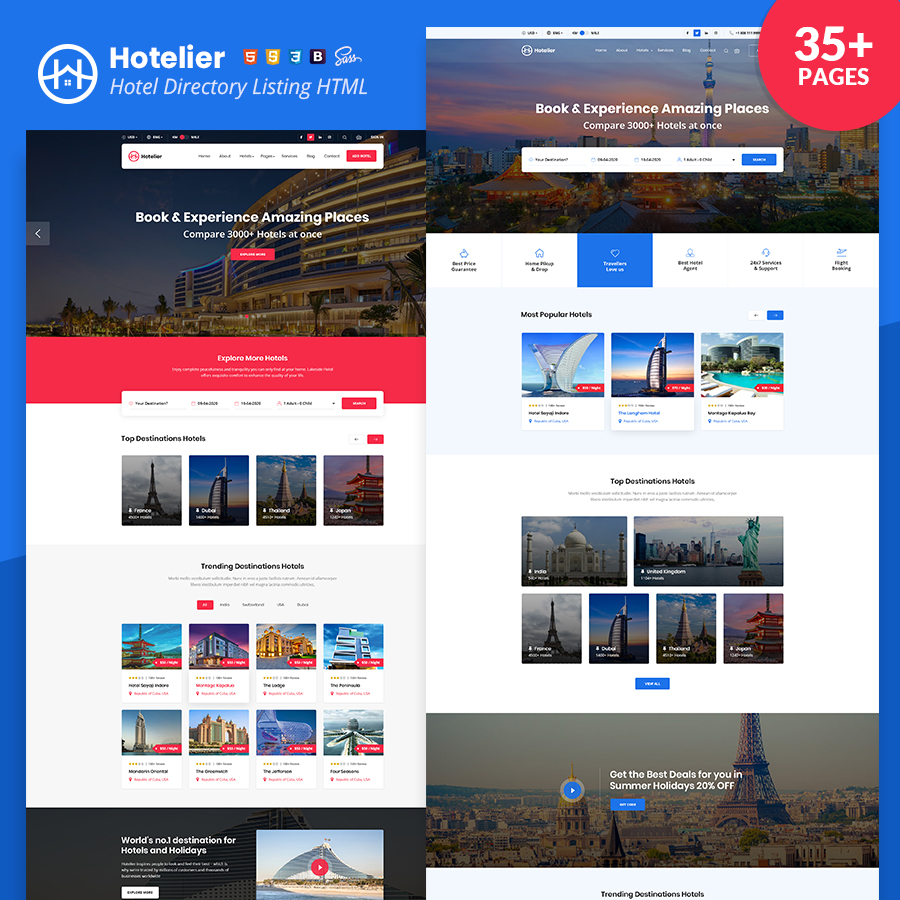The image showcases a template for "Hoteller: Hotel Directory Listings," an HTML-based framework designed for creating comprehensive hotel directories. The template boasts over 35 pages, meticulously crafted to enhance user experience when exploring accommodation options. The highlighted features of the template include the ability to book and experience a variety of exceptional places, a tool to compare over 3,000 hotels simultaneously, and sections for exploring more hotel options. Key categories within the directory template are "Trending Destination Hotels," "Top Destination Hotels," and "Most Popular Hotels." Additionally, it promotes exclusive offers, such as a 20% discount for summer holidays.

Visually, the template is displayed against a blue background, with two sample pages of the website overlaying this backdrop. These pages provide a glimpse into its sleek design and user-friendly layout. "Hoteller: Hotel Directory Listings" serves as a ready-made HTML solution for building a hotel directory website, enabling users to easily input their content and images to create an attractive and functional directory.